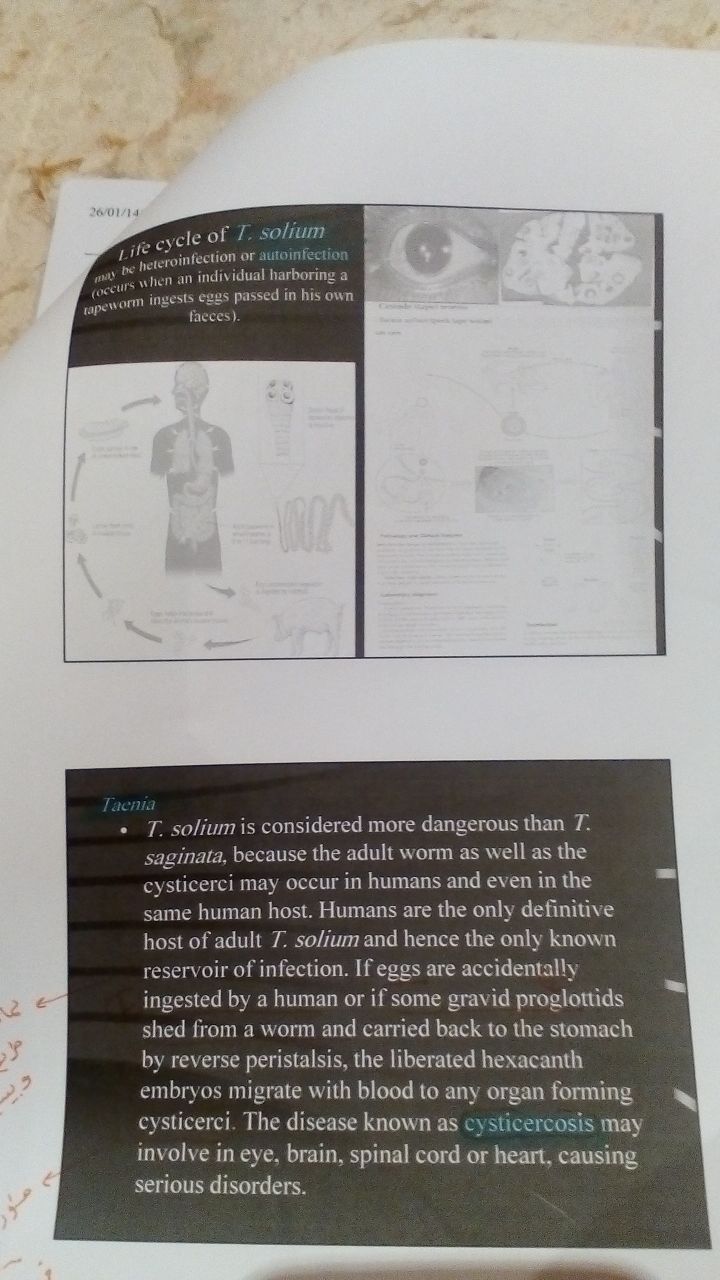The image depicts a printed piece of paper, which appears somewhat folded and lies on a white and brown table or countertop. The top left corner of the paper is noticeably curled. The content of the paper is extremely faded, making it challenging to discern, but several detailed observations can be made. At the very top right, there are images related to the life cycle of the T. soleum tapeworm, including visuals of a human eye, a brain scan, and a diagram displaying internal human organs. Additionally, the top left features depictions of people with symptoms from tapeworm infections. In particular, the text near these images details the lifecycle of T. soleum, explaining concepts such as hetero infection and auto infection, notably the process where a person harboring a tapeworm might ingest eggs from their own feces. Below these illustrations and descriptions, a black box with white text explains the medical complexity of T. soleum infections. It highlights the dangers posed by T. soleum, emphasizing that humans are the definitive hosts and the sole reservoirs of the infection. The text outlines severe health complications that can arise if eggs are ingested, leading to the formation of cystocerci in vital organs like the eye, brain, spinal cord, and heart, thereby causing serious disorders.